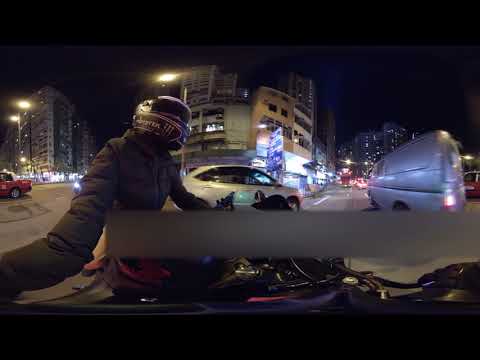The nighttime city street scene captures a panoramic view from the perspective of a motorcyclist wearing a black helmet and thick winter jacket on a dark-colored motorcycle with light pink or purplish accents. The rider is turned slightly to the side, possibly holding a camera or a selfie stick. The scene is bustling with activity as various vehicles, including a white car beside the motorcycle and other cars like a van, sedan, and truck, maneuver through a large intersection. In the background, tall city buildings and a rounded corner store stand brightly lit, while streetlights illuminate the road. The far distance reveals the brake lights of other cars, adding depth to the image. A thin black line runs horizontally across both the top and bottom of the image, and a blurred rectangle appears just below the center, obscuring part of the scene.